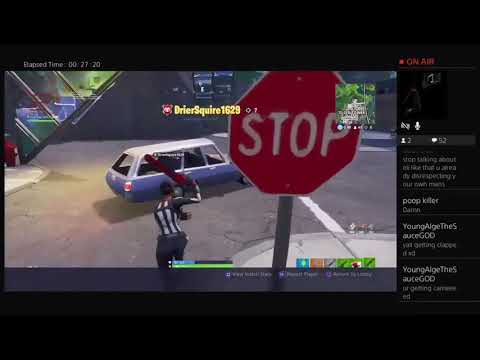This image is a still shot from a video game, appearing as a square digital scene. Prominently, a giant stop sign is centered towards the right. On the left, a character dressed in a referee outfit chases a station wagon-like car, which is blue with a white top. The background features some buildings, giving a street scene atmosphere. Notable colors in the image are dark red, black, gray, blue, white, green, and orange. The screen name "Brief Squire 1629" is displayed in white text near the top of the image, while the bottom part contains small icons that are too difficult to discern. The image is framed with black rectangles at the top and bottom.